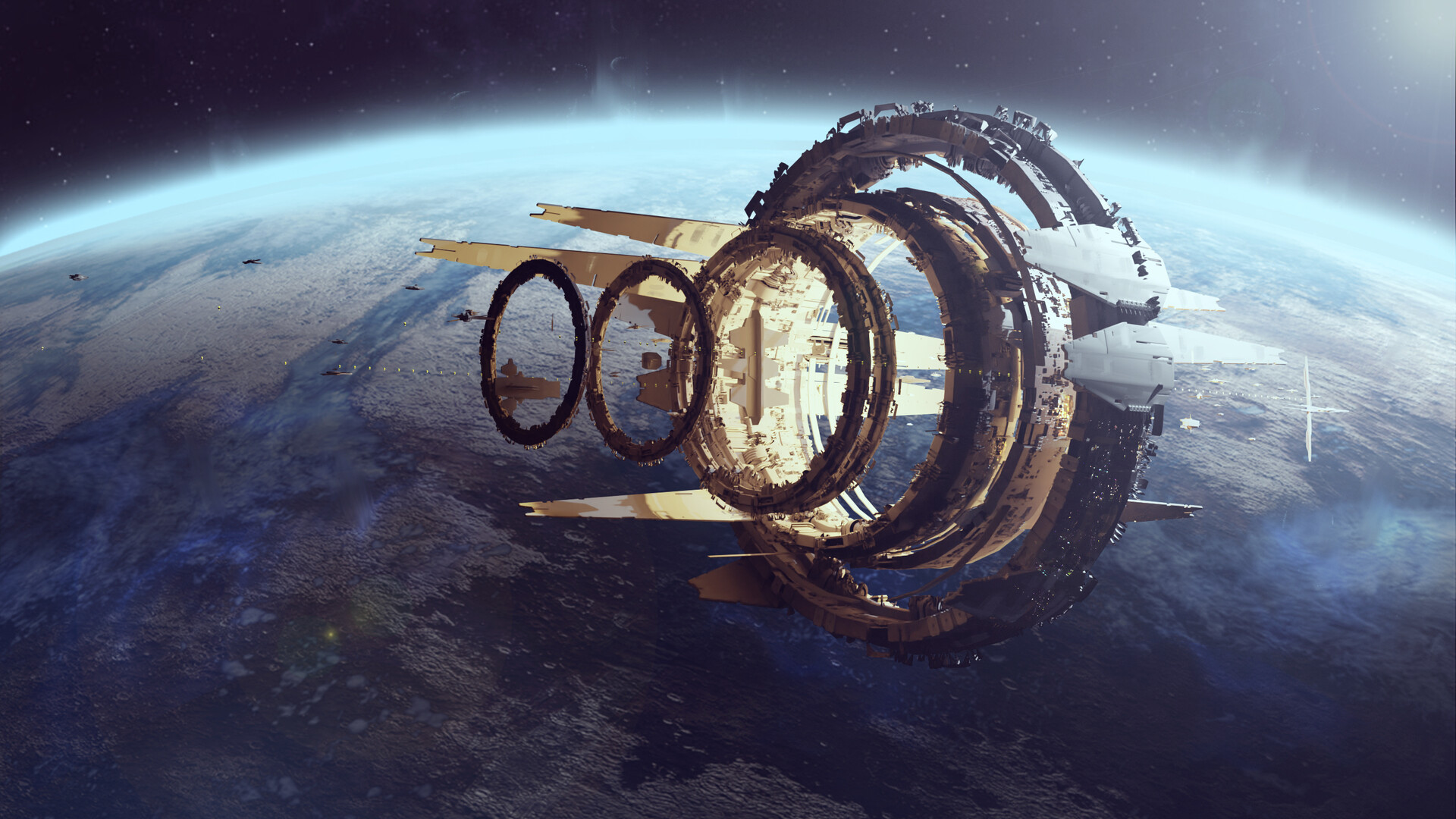The image showcases an intricate and sophisticated space station, possibly an AI-generated artwork, set against the stunning backdrop of Earth from space. The space station, predominantly black with accents of beige, tan, and gray, occupies the central portion of the image and tilts slightly towards Earth. The station's design includes multiple rings that seem to be stacked, connected by long pillars, and other circular and metal-like structures extending from its sides. 

Earth dominates the lower two-thirds of the background, exhibiting its curvature along with visible landmasses and oceans. A striking thin blue glow traces the planet's upper edge, enhancing the ethereal quality of the scene. The top right corner hints at a light source, inferred to be the sun, illuminating the station and casting shadows on parts of it while remaining out of the frame. The upper portion of the image features the dark expanse of outer space, dotted with stars, contrasting with the illuminated Earth below, making for a visually captivating and detailed portrayal of a sci-fi-esque setting.